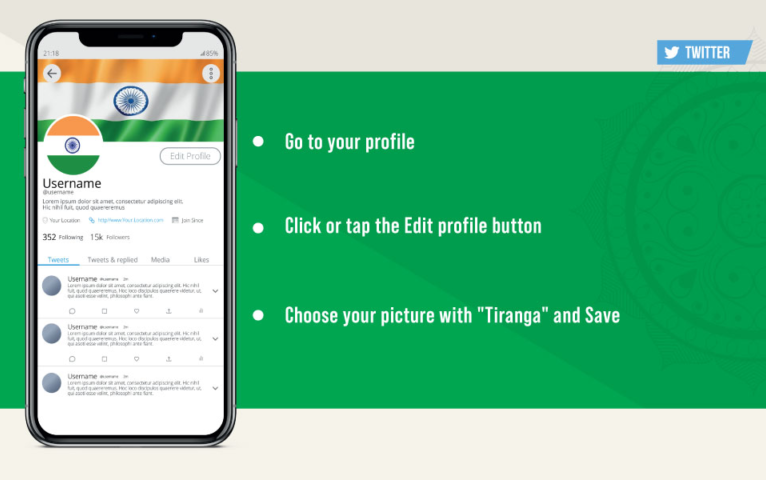This infographic features an instructional guide on a largely green background, complemented by gray banners at the top and bottom. Central to the design is the image of a cell phone displaying a Twitter page on its screen. The phone shows visible bezels and buttons, focusing on the front view.

The displayed Twitter profile includes an avatar featuring an orange horizontal stripe, a white stripe, and a green stripe with a blue circle containing a blue sun in the middle. The username field is generic, indicative of a placeholder or mock-up.

Adjacent to the phone image, white text on the green background offers clear instructions in three bullet points:
1. Go to your profile.
2. Click or tap the "Edit Profile" button.
3. Choose your picture with Tiranga and save.

"Tiranga" is highlighted and spelled as T-I-R-A-N-G-A. The familiar Twitter logo, a bird with the text "Twitter," is prominently placed in the top right-hand corner of the image.